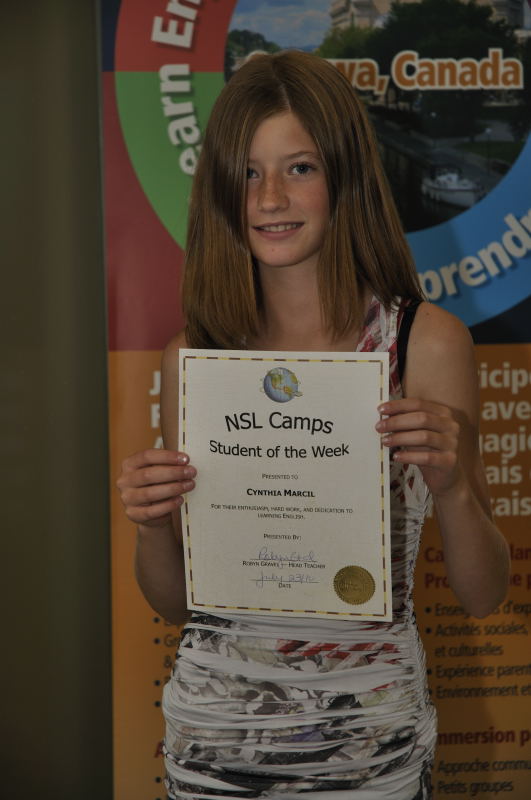In the image, a young girl, around 13 or 14 years old with red hair, stands directly in the center, holding a certificate prominently toward the camera. The certificate reads "NSL Camp Student of the Week," awarded to Cynthia Marcell for her enthusiasm, hard work, and dedication to learning English, presented by her home teacher, though the teacher's name isn't legibly visible. The certificate also features a globe at the top and is adorned with various colors, including brown, orange, red, green, blue, purple, light blue, and gold. The background is an off-gray or brownish hue with a partially obscured sign or poster. The setting appears to be indoors, likely during an award presentation, possibly in Ottawa, Canada, suggested to be related to a special convention for kids, dated July 23rd, though the year is not specified.